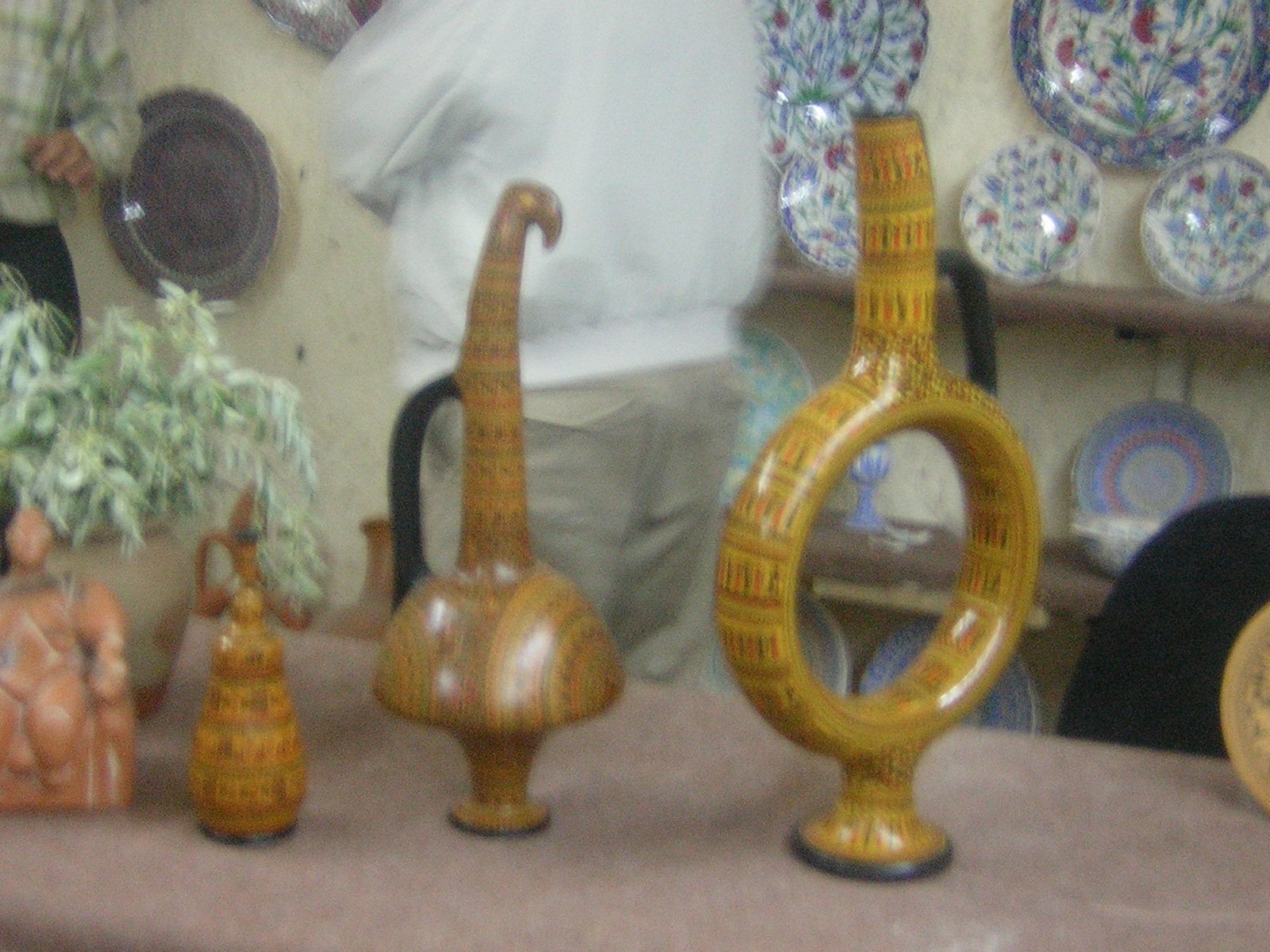The image depicts a slightly blurry, out-of-focus scene that appears to be from a collectibles store or an exhibit of artifacts. A narrow, reddish-brown table in the foreground holds four sculptures, each distinctive in shape and material. On the left, there's a tiny, terracotta-like Buddha statue. Next to it stands a gourd-shaped sculpture with a handle, adorned with a painted pattern. The third piece, crafted from wood, resembles a flamingo with a tall neck and rounded body, standing on a narrow base. The fourth sculpture is a large circular piece with a long neck, decorated with repeating painted patterns both inside and out. To the left, a houseplant with green and white leaves sits in a tan-colored stone pot.

In the background, a light beige wall hosts narrow wooden shelves lined with white ceramic plates featuring blue and red designs. Two individuals are partially visible: one, in the center, wears a white jacket and tan khaki pants; another, further back, wears a green plaid shirt and blue pants, standing in front of a large blue ceramic plate displayed on the wall. The image, taken indoors, captures a sense of antiquity and cultural richness, despite its grainy and unclear quality.